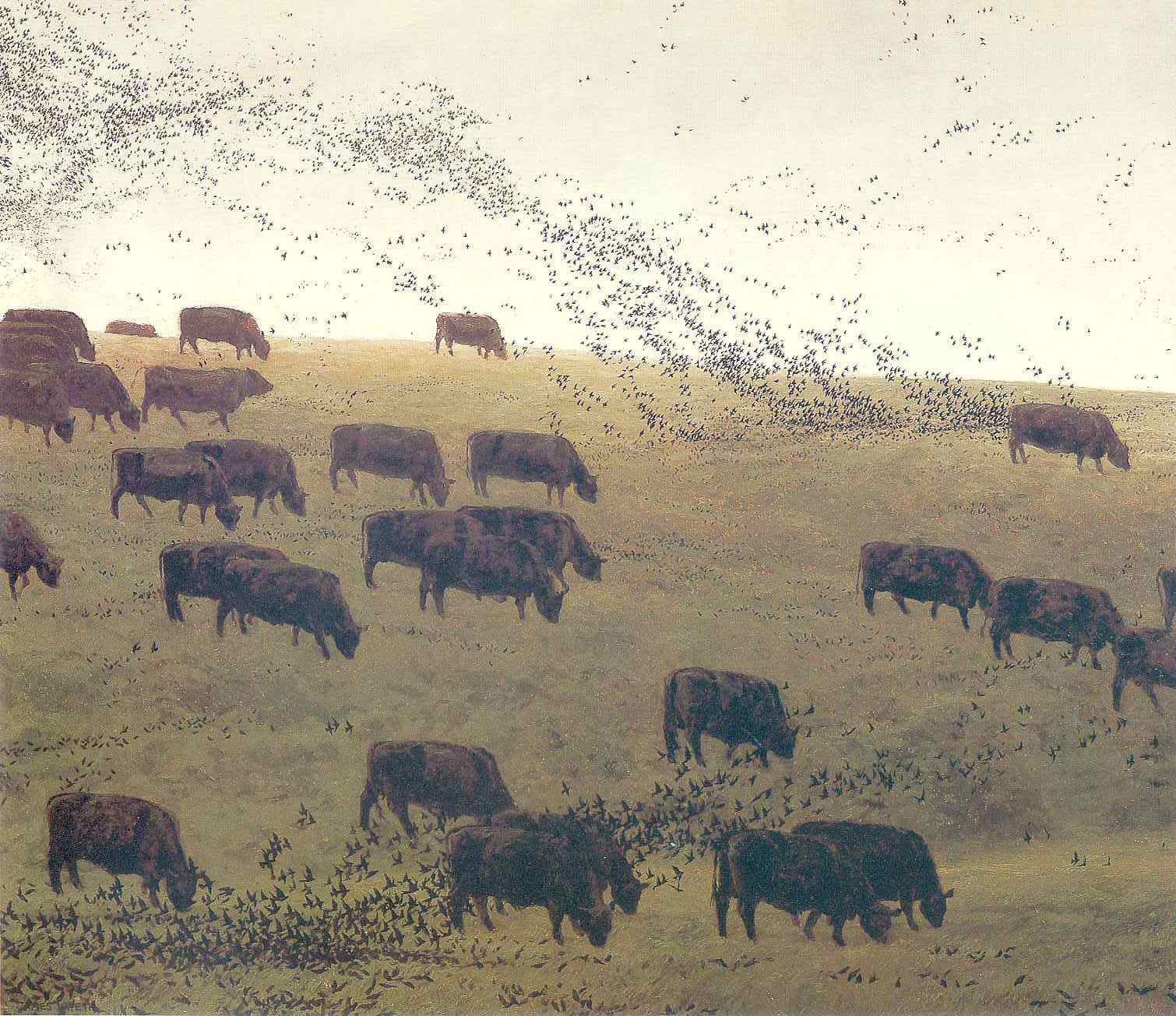This outdoor painting showcases a serene pastoral scene of approximately twenty cows, primarily brown with some darker hues, grazing on a gently sloping pasture. The cows are scattered throughout the grassy field, their heads mostly bowed as they feed on the greenery. Among them, one cow stands out with its head raised. The field itself is a patchwork of greenish-yellow tones, adding subtle variation to the landscape. The ambiance is animated further by flocks of small, black birds; some are perched on the grass, while others ascend into the air, disturbed by the grazing cattle. The sky is a moody, cloudy gray, contrasting with the earthy hues of the field and cattle. This painting captures a moment of natural harmony, devoid of text, emphasizing the tranquil coexistence of livestock and wildlife.